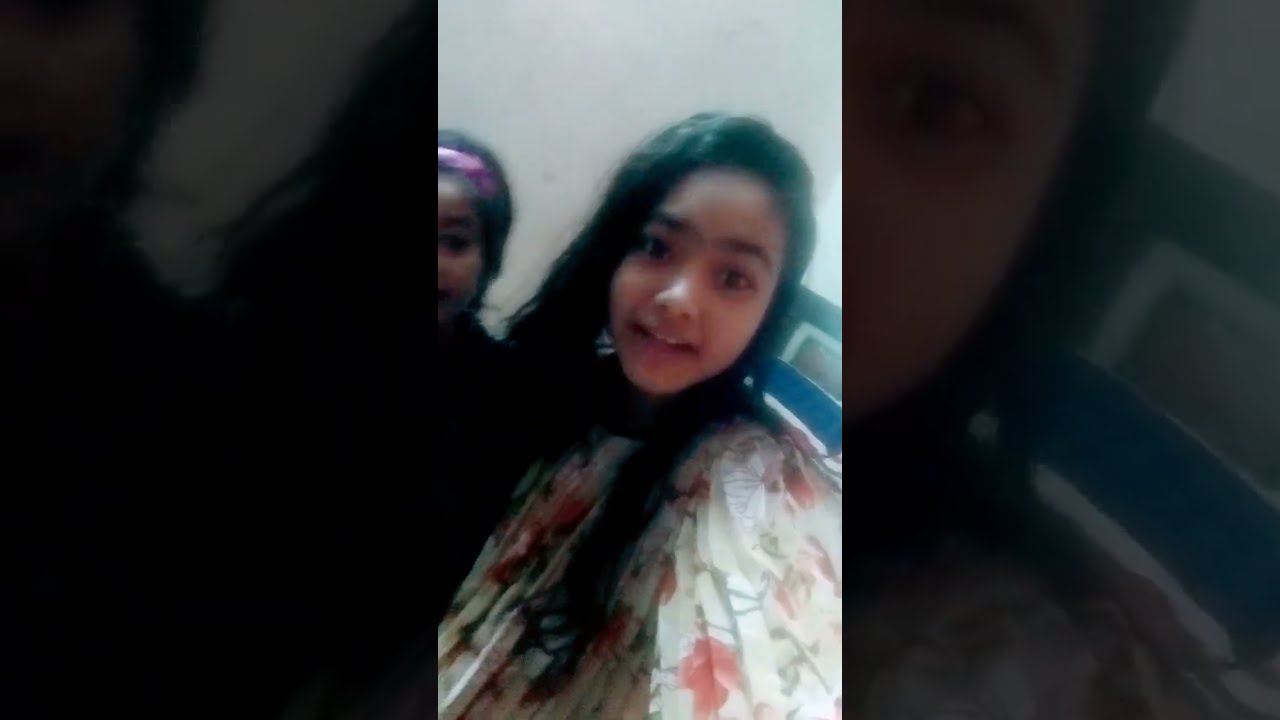In this slightly grainy and blurred image, we see two young girls, likely aged 12 to 14, who appear to be of Asian or Hispanic descent, each with light brown skin. The photo, taken at an angle from about mid-waist up, depicts the girls emerging from the lower left-hand corner of the frame. The girl closest to the camera has long, straight black hair and is wearing a white blouse adorned with orange-pink flowers, characterized by its flouncy appearance. She is looking directly at the camera with an open mouth, revealing the top of her teeth, and her right hand raised with the palm facing outward, as if she is waving or signaling stop. Just behind her, to the left, stands another girl with pulled-back straight dark brown hair held by a bandana. Her eyebrows are creased upward in the center, and she wears a grimacing smile. Both girls have their hands near their chins, palm up, with the girl in front using her left hand and the girl in the back her right.

The photo has been enlarged and darkened to create a thick border on the left and right sides of the main image, featuring zoomed-in sections of the girls' faces. The overhead light source causes a noticeable shine on the tops of their heads and foreheads, adding to the portrait's overall effect. The entire picture has a diagonal tilt clockwise, adding to the dynamic composition.